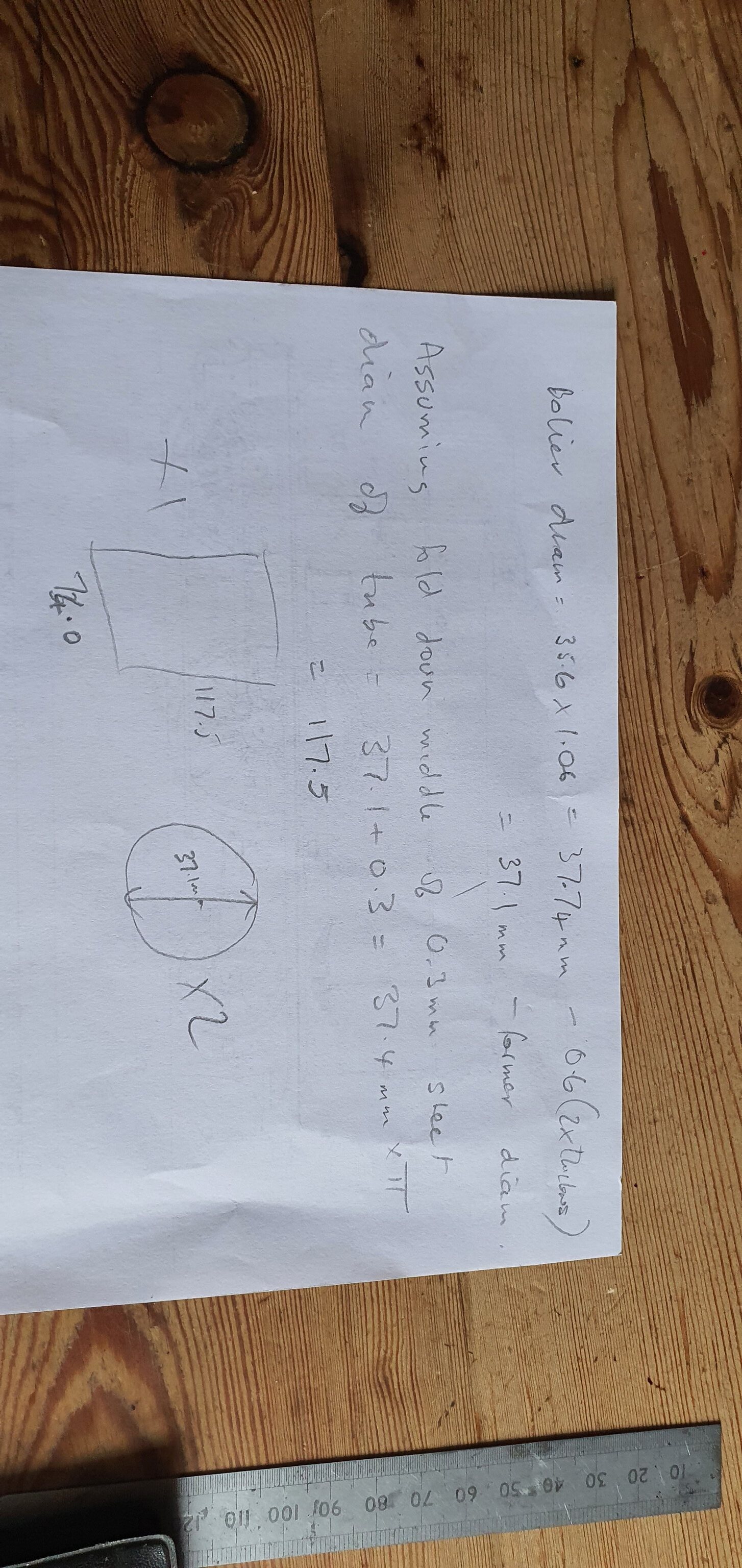The image displays a detailed scene of a wooden table with a light brown grain interspersed with dark knots. Positioned sideways, the primary subject—a piece of paper—is predominantly covering the frame, with its bottom edge on the left and top edge on the right. On this paper, written in scribbled black ink, are a series of mathematical equations and figures. Among these, a rectangle labeled "X1" with specified side measurements and a circle labeled "X2" indicating a 37-inch diameter stand out. The equations are difficult to decipher due to poor penmanship. At the bottom of the image, also oriented sideways, is a metal ruler, partly obscured within a black case or holder. This arrangement of items captures a moment of study or problem-solving, framed by the rustic charm of the wooden tabletop.